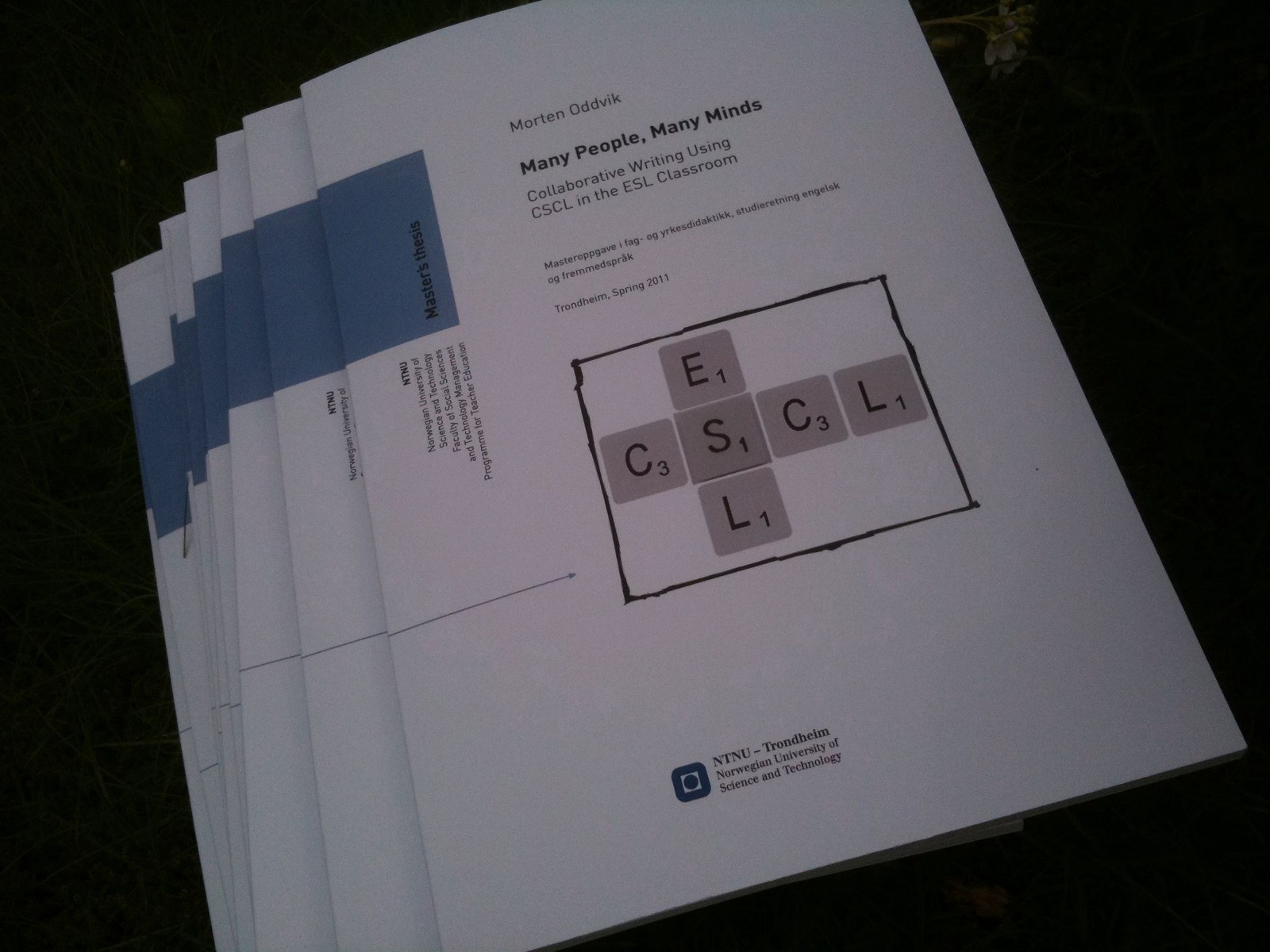The image depicts a detailed view of seven white booklets stacked on top of each other on a black tablecloth. Prominently titled "Many People, Many Minds: Collaborative Writing Using CSCL in the ESL Classroom," the booklet's cover features black text. Underneath this title, the authorship attributed to Morten Odvik is visible. A striking design element includes letters reminiscent of Scrabble tiles, arranged to form "CSCL" in a horizontal line, intersecting with "ESL" vertically, all within a black square. At the bottom of the booklet, it states "NTNU Trondheim, Norwegian University of Science and Technology." Additionally, each booklet displays a small blue square on the top left corner, marked with "Master's Thesis" in white text. The image’s background, entirely black, contrasts with the booklets, enhancing their visibility and detail.